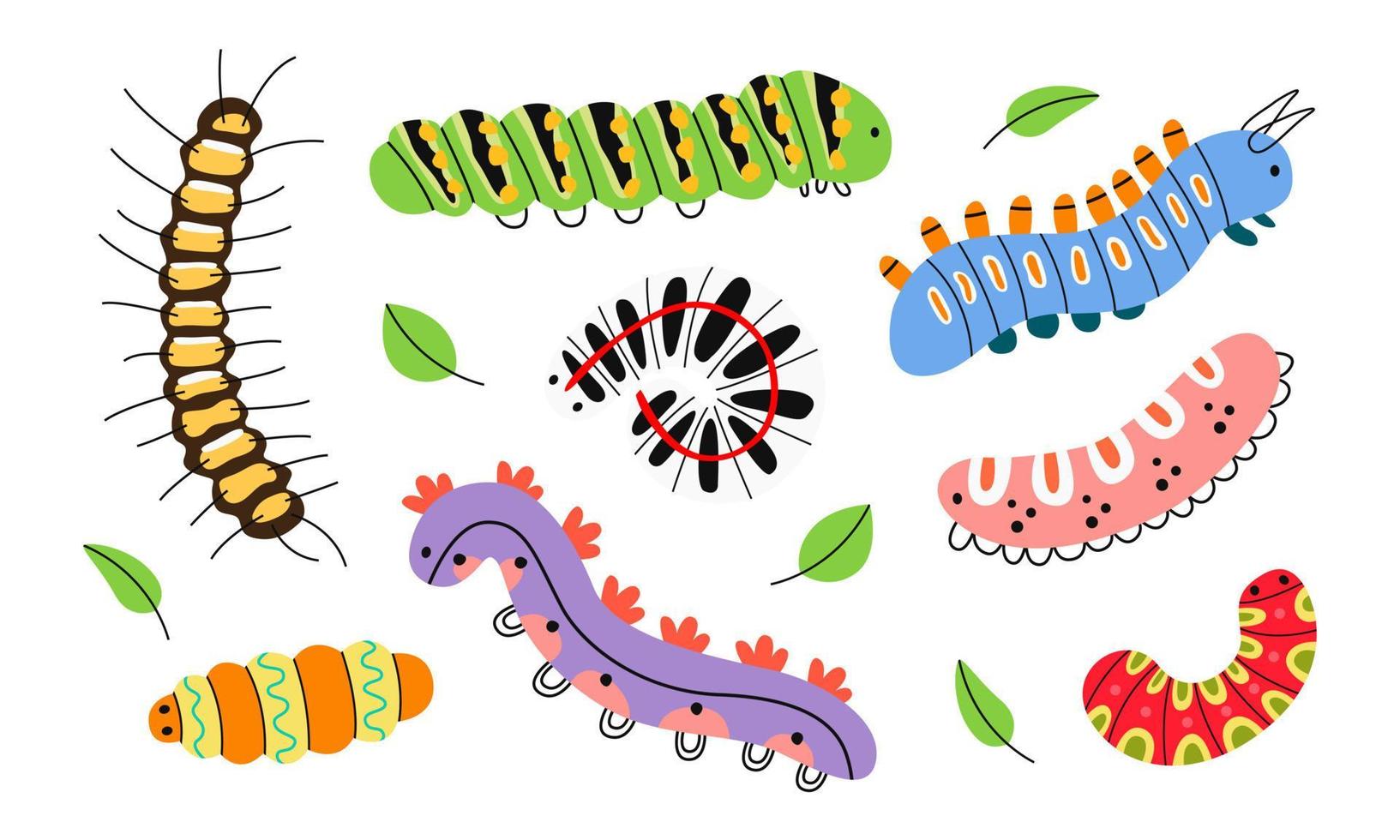This image showcases a charming, cartoonish illustration of various colorful caterpillars against a solid white background. Starting from the top and moving clockwise, the details are as follows:

1. A green caterpillar adorned with black stripes and yellow dots.
2. To the right, a blue caterpillar featuring orange dots and stripes along its back.
3. Below is a pink caterpillar with orange stripes and small black feet.
4. Further down, there is a red caterpillar with decorative green and yellow dots and stripes.
5. In the middle, a long purple caterpillar with spiny orange protrusions and tiny black feet can be seen.
6. To the left, a short caterpillar viewed from above, characterized by alternating orange and yellow segments with wiggly blue lines.
7. A larger, brown, segmented caterpillar is situated up and to the left, each segment containing yellow and white patterns.

Additionally, there are five green cartoon leaves scattered between the caterpillars. The central background features a pattern of lines and stripes with a notable red line running through it, adding to the playful and whimsical nature of the image.